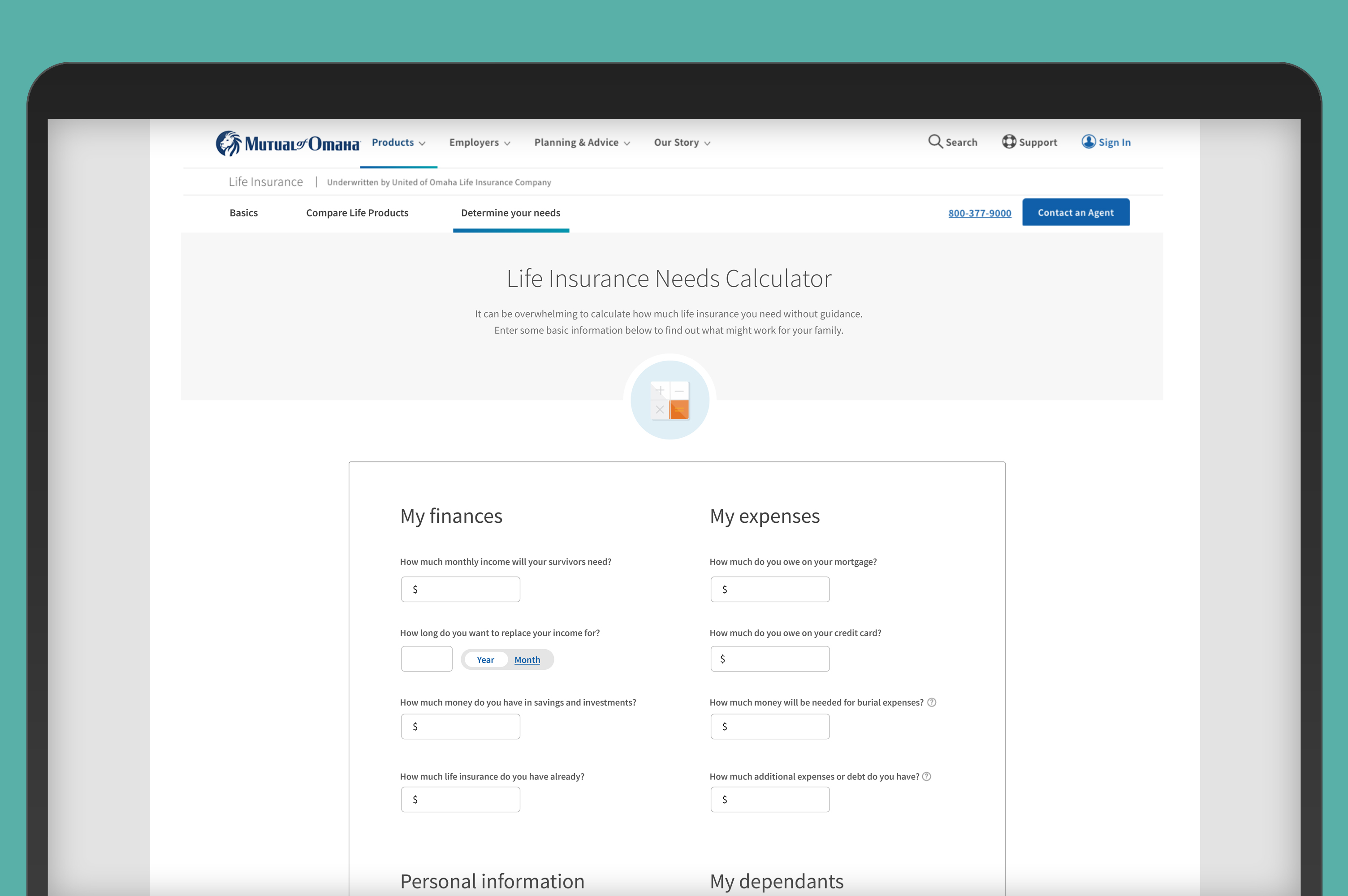This image features a detailed view of Mutual of Omaha's website displayed on a computer monitor. The monitor has a black outline, and the webpage has a predominantly white background. At the top left, the Mutual of Omaha logo is prominently visible in blue, featuring their recognizable stylized insignia to the left of the textual logo. To the right of the logo, a navigation menu includes links titled "Products," "Employment," an unreadable link, "Planning and Advice," and "Our Story." Moving further right, there are icons and text for "Search" (marked with a magnifying glass), "Support" (indicated with a globe icon), and "Sign In" (represented with a person icon). Most of the text in the menu is in shades of grey to black, except for "Sign In" and "Products," which are highlighted in blue, indicating the currently selected tab.

The "Products" page is displayed, offering options related to Life Insurance. Below the main logo, the term "Life Insurance" reappears, accompanied by some unreadable text to the right. The page provides links to "Basics," "Compare Life Products," and "Determine Your Needs," with "Determine Your Needs" underlined, highlighting the active tab. Beside these links, there is a blue box with white text featuring a clickable 800 number for contacting an agent.

Under this section, the page presents a "Life Insurance Needs Calculator" heading in grey, accompanied by a small, non-clickable calculator icon. This is followed by an interactive calculator interface where users can input data under several categories, including "My Finances," "Personal Information," "My Expenses," and "My Dependents." Each category has four input boxes, with headings that are too small to decipher, except for "Personal Information" and "My Dependents," whose input boxes may require scrolling to view entirely.